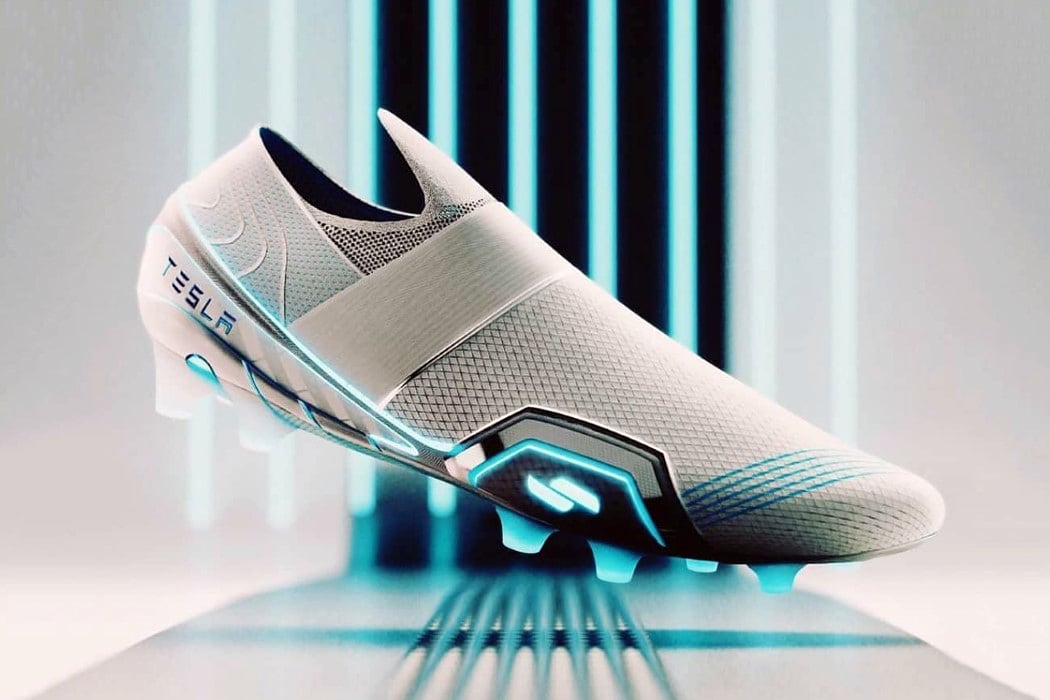The image features a hyper-modern, futuristic Tesla sneaker displayed in a pristine, minimalist setting. The horizontally-oriented, computer-generated product image showcases the sneaker, which is predominantly white with striking neon sky blue accents. The sneaker, which fills the frame, is made from a sophisticated, lightweight material that resembles a smooth, woven fabric. Notably, it lacks traditional shoelaces, instead opting for an elastic strip over the top, enhancing its sleek and seamless design. 

The shoe is positioned with its heel to the left and toe to the right, appearing almost slipper-like in its smoothness. The tongue departs from standard shoe design, further contributing to the modern aesthetic. The sole features blue highlights, and the Tesla logo is prominently displayed along the heel and side. The sneaker is perched on a small stand, adding to its visual prominence.

The setting amplifies the futuristic vibe: the background is a white room with a black vanishing point intersected by neon blue lines, creating a sense of depth and motion. Rectangular slots, similarly white and neon blue, complement the high-tech theme. Additionally, blue lines extend from the foreground to the background, further accentuating the impression of speed and innovation. Beneath the shoe, plastic cleats suggest a versatile design, potentially suitable for soccer or other athletic endeavors. Overall, this Tesla sneaker epitomizes cutting-edge design, merging style with advanced functionality.